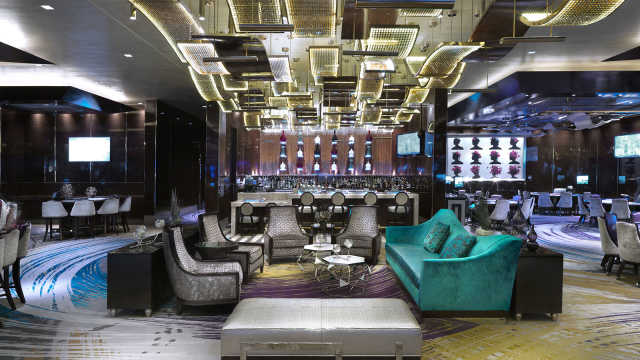The image depicts a lavish and modern bar, reminiscent of an upscale establishment located in a high-end hotel or VIP section. On the left side of the image, large tables are surrounded by ornate chairs, upholstered in white pearl fabric. In the center, there are four lower chairs in the same opulent fabric and two small, uniquely-shaped tables with one appearing to be a white rectangular footrest or papasan. Adjacent to these chairs is a bold turquoise-teal-blue couch. 

Dominating the background is a stylish bar area, featuring arm-free bar stools, also lined in the ornate white pearl fabric, and stocked with a wide assortment of alcohol. To the right of the bar, more circular tables are surrounded by matching ornate chairs. 

The establishment is accentuated by wavy ceiling panels emitting light in various shades of gold and browns, creating a warm glow. The ceiling panels are diverse in shape and size, enhancing the space's sophisticated ambiance. The floor below transitions beautifully from white and blue wave patterns to gold and brown waves, with hints of burgundy near the center. Additional features include a vibrant emerald green couch on the right and silver, sparkly chairs placed throughout the room. TVs are visible in both the top left and top right corners of the image, contributing to the overall contemporary and luxurious setting.